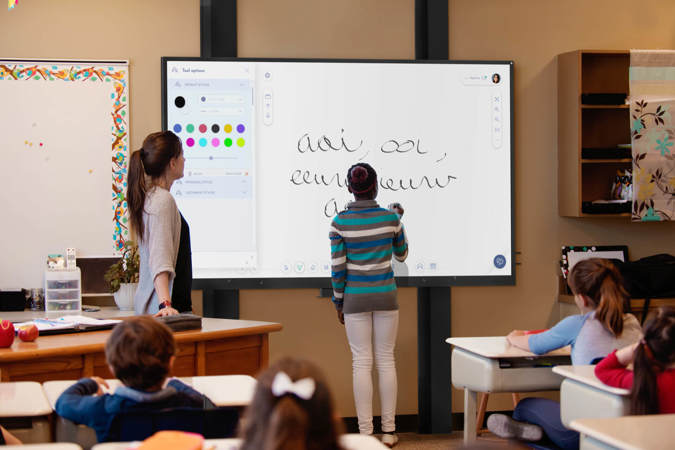This photograph captures a modern classroom scene with a group of elementary school children, approximately fourth or fifth grade age. The children are seated at white desks, their attention focused on a large electronic whiteboard at the front of the room. In the foreground, the backs of four children’s heads are visible as they sit at their desks, intent on the activity at the board. The children, three girls and one boy, all appear to be Caucasian with dark hair.

At the front of the room stands an African American girl about 10 or 11 years old, dressed in white jeans and a striped long-sleeved sweater in shades of blue, white, and tan. Her hair is neatly styled in a bun. She is writing in what seems to be French on the large electronic whiteboard, which dominates the front wall. The board is massive, bigger than the girl herself, and appears to be more high-tech than a traditional whiteboard.

To the left of the young girl, a female teacher stands in profile, observing the student's work. The teacher appears to be in her 30s, with a long brown ponytail, and is wearing a cream or beige-colored sweater over a black shirt. She is also sporting a red and white watch and is seen leaning her hand against a desk, her gaze fixed on the board. The classroom environment is well-lit, clean, and exudes a sense of comfort and order, with a light brown wall on display to the left of the electronic whiteboard, including a traditional whiteboard affixed to it.